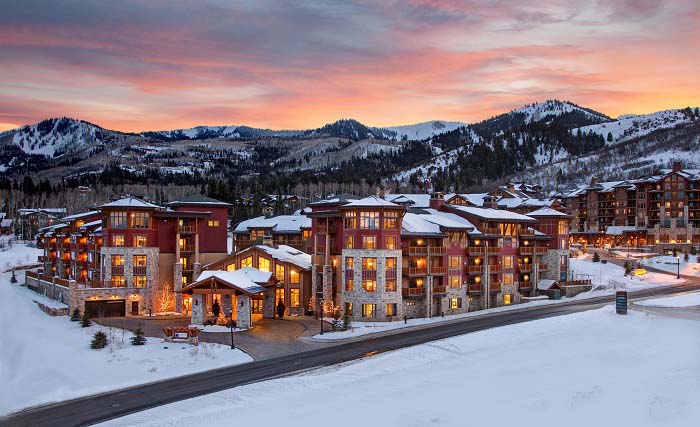This photo captures a serene winter evening at a large, well-lit mountain resort nestled under snow-covered mountains. The scene showcases a sunset casting a warm orange and yellow glow across the sky, which contrasts beautifully with the grayish-blue clouds. The resort complex, constructed with a stone bottom half and brick-red top half, stands prominently amidst the snowy setting. The windows of the resort are warmly lit, suggesting a cozy interior. 

In the foreground, a roundabout driveway with an overhang leads to the main entrance, which is neatly connected to a small paved road running from the bottom left to the middle right of the image. Sidewalks and pathways around the resort are cleared of snow, emphasizing the meticulous upkeep of the premises. Further roads can be seen stretching into the distance, likely leading to other buildings within the resort complex. 

The entire area is blanketed in snow, covering the ground and rooftops alike. Snow-covered hills dotted with evergreen trees rise behind the resort, while the more distant mountains add to the majestic backdrop. Despite the absence of people or moving vehicles, the illuminated buildings and cleared pathways suggest a bustling activity within, possibly with guests enjoying the ski slopes or relaxing indoors at this seemingly fancy ski lodge.